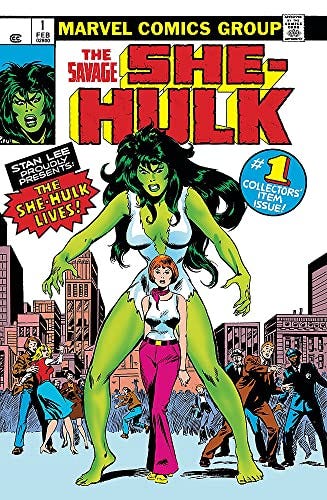The image is the front cover of a classic comic book, likely from the 1960s or 70s, titled "The Savage She-Hulk." At the top, the header reads "Marvel Comics Group" in yellow letters on a black background. Beneath this, in bold red letters with a yellow 3D effect, is the title "The Savage She-Hulk." Adjacent to the title is a small image of She-Hulk's face, showcasing her green complexion, thick black hair, arched eyebrows, and large lips.

Just below the title, in smaller blue letters, it proudly announces "Number One Collector's Item Issue." To the left, a black and white banner states, "Stan Lee proudly presents The She-Hulk Lives!"

Dominating the cover is the main illustration featuring the She-Hulk, who towers over everyone else in the scene. She is depicted with a powerful and imposing physique, green skin, and thick, flowing black hair. She is dressed in a white outfit resembling a bikini, exuding both strength and presence. Before her is a smaller woman, dressed in purple bell-bottoms, a white shirt, and a purple scarf, with her short red bob haircut and bangs clearly visible. This woman appears almost vulnerable next to the She-Hulk.

In the background, there is a cityscape with four visibly frightened people—a cop, a man, a woman, and another man—staring up at She-Hulk in alarm. The urban setting amplifies the dramatic, chaotic scene unfolding on the comic book cover.